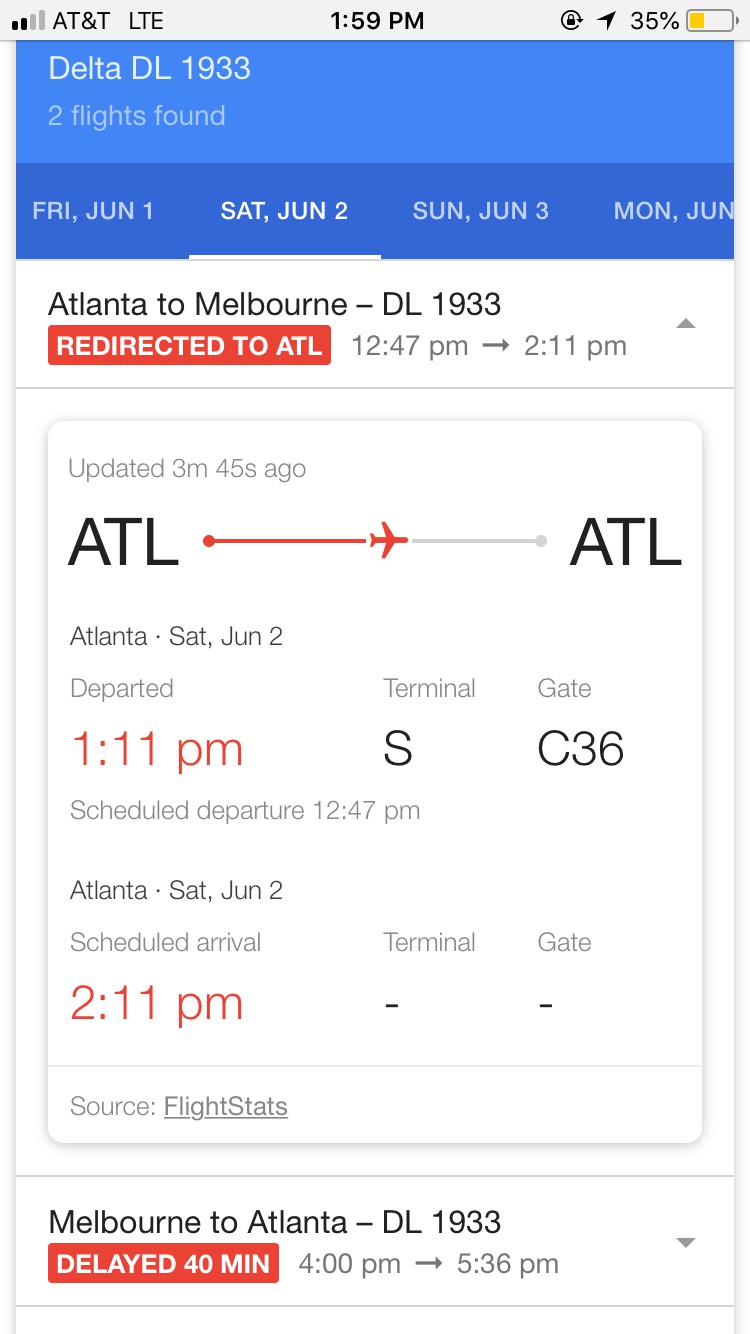This is a detailed caption describing the contents of a screenshot in portrait mode. The image captures various sections of a flight tracking application or website, complete with date-specific information, flight status, and relevant logistics. 

In the upper left corner, there is a gray strip indicating the cellular carrier "AT&T" on the left. The time "1:59 p.m." is displayed prominently in the center, with the battery level at 35% on the right. Below this is a light blue section indicating the flight number "Delta DL 1933." However, the light blue text on the light blue background makes it difficult to read the “Two flights found” notification beneath it.

The subsequent row with a blue background has several tab headings for different dates: "Friday, June 1st," "Saturday, June 2nd," "Sunday, June 3rd," and "Monday, June 4th," with the user needing to scroll right to see more dates. The tab for "Saturday, June 2nd" is bold and underlined, indicating that this is the active selection.

The section below features a white background and provides specific flight details for “Atlanta Melbourne DL 1933.” It has a large red button stating “redirected to Atlanta ATL” with a timeframe of "12:47 p.m. to 2:11 p.m." and an option to view more details. An update note follows, mentioning that this information was updated three minutes and 45 seconds ago. It seems the flight may have been rerouted back to Atlanta, as indicated by multiple mentions of Atlanta. 

Additional details follow:
- Flight from Atlanta on Saturday, June 2nd, departed at 1:11 p.m. from Terminal S, Gate C36. The scheduled departure was initially at 12:47 p.m.
- Scheduled arrival in Atlanta on the same day at 2:11 p.m.

The following flight segment from Melbourne to Atlanta for "Delta DL 1933" shows a delay of 40 minutes, with the new timings being 4:00 p.m. to 5:36 p.m.

Overall, the image captures a comprehensive overview of the flight's schedule, status updates, and logistical information, making it clear that the flight has experienced some delays and redirections.